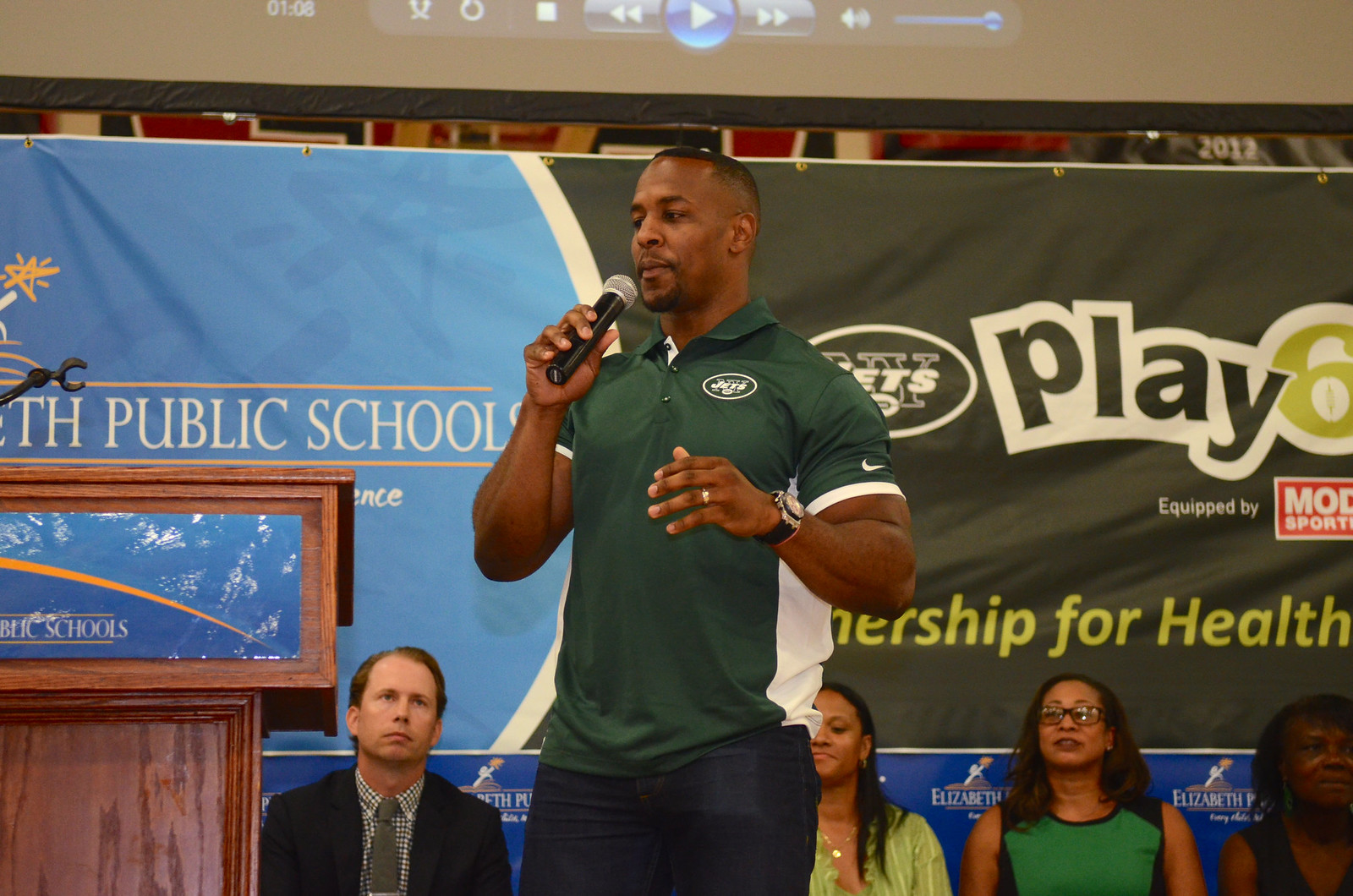In this photograph, an athletic African-American man, likely in his late 20s to early 30s, is depicted speaking into a black microphone. He stands confidently at a three-quarter angle facing left, dressed in a tight, short-sleeved green polo shirt with a white stripe down the side, a white Nike logo on the sleeve, and a Jets logo on the chest. His attire is completed with dark blue jeans. His hair is closely cropped, and he has a short goatee.

He is positioned in front of a large, divided banner. The left side of the banner, characterized by a blue background, partially displays the words "Public Schools" and features a small section of an additional logo. The right side of the banner, set against a dark green backdrop, prominently showcases the word "PLAY" in large, green letters heavily outlined in white alongside the Jets logo, and the phrase "Leadership for Health."

To his left, there is a wooden podium, and seated behind him are several individuals. An older white man in a suit and tie is sitting to the man's left, while to his right are three African-American women: one in a light green blouse, another in a sleeveless green shirt trimmed with black and wearing glasses, and the third partially cut off by the photograph, dressed in black. Above, a projector screen with visible playback controls suggests a multimedia presentation is part of the event. The setting appears to be a public school, possibly for a 'Jets Play 60' event aimed at promoting health and fitness.